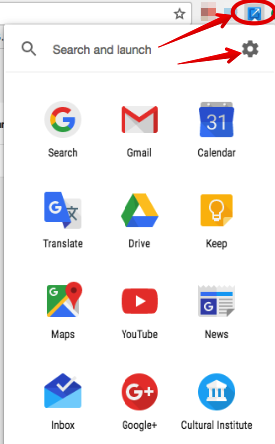In this image, we see a detailed screenshot of an Android device displaying numerous apps prominently. The apps visible on the screen include Google Search, Gmail, Calendar, Translate, Drive, Keep, Maps, YouTube, News, Inbox, Google+, and Cultural Institute. The interface is designed within a white background, accentuated by vibrant colors such as green, yellow, blue, and red, typically associated with Google's branding. Two arrows are notably present in the image; one is pointing towards a settings button, indicating its location, while the other arrow directs attention towards the top right corner of the screen. Additionally, there's a search field at the top labeled "Search and launch," facilitating easy navigation and access.